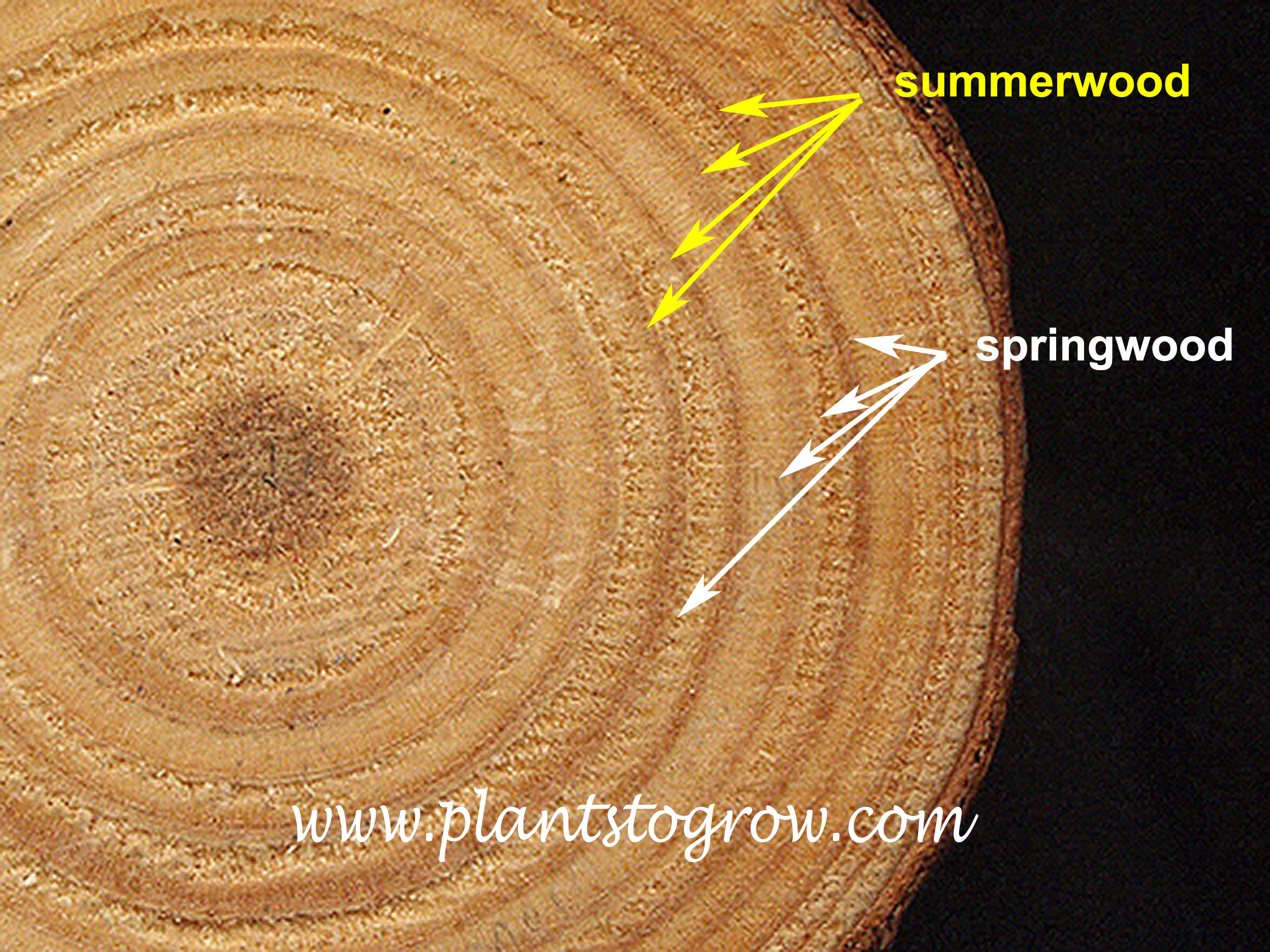The image is a detailed close-up painting of a tree stump, showcasing the intricate rings that signify its age. The stump has been cut in half and is zoomed in just enough that the entire stump is not visible, with the left side cut off and the right side revealing its rounded edge. The central part of the stump is a darker brown dot, transitioning into various shades of brown and beige towards the outer rings. The background to the right side of the image is black, which accentuates the vibrant yellow and white text overlaying the image. At the top right corner, the words "summer wood" are written in yellow font, with four yellow arrows pointing to different areas on the stump. Below that, the words "spring wood" are written in white, accompanied by four white arrows indicating other parts of the stump. At the very bottom of the image, in white cursive lettering, is the URL "www.plants2grow.com," possibly suggesting that the image is promoting this website. The overall color scheme prominently features shades of brown, beige, white, and a vibrant yellow.